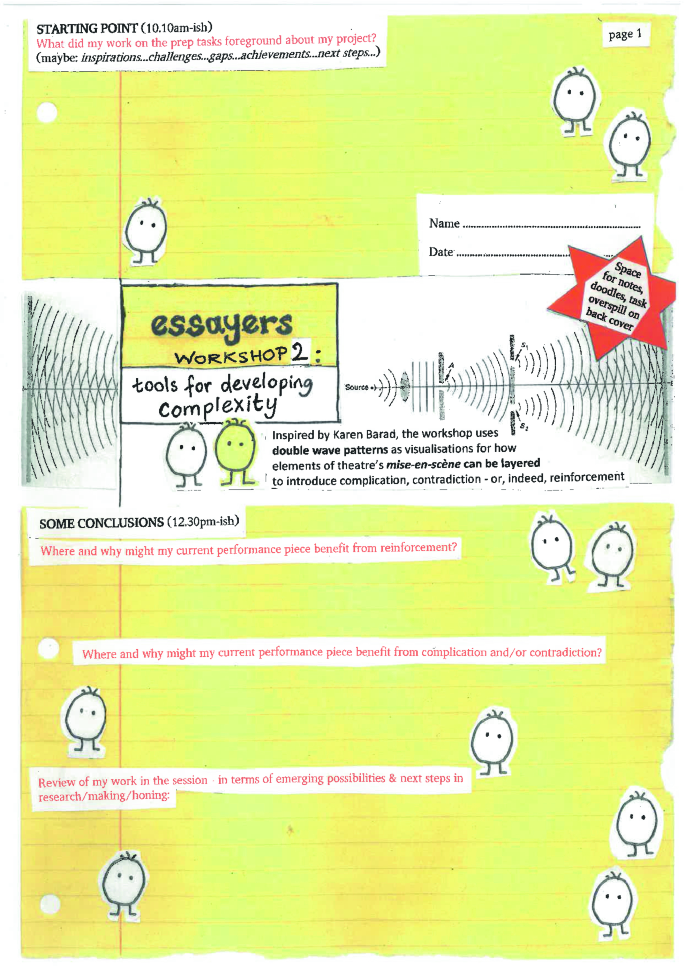The image is a detailed drawing resembling a yellow lined sheet of notebook paper, filled with considerable text and whimsical illustrations. Dominating the center is the title "Essayers Workshop 2: Tools for Developing Complexity." The background, a soft yellow, is sprinkled with round, stick-figure-like characters with big eyes, two legs, and three tiny tufts of hair. These characters are predominantly white, with one in a very light green.

The page features multiple sections of text, including a portion inspired by Karen Barad, emphasizing the use of double-weave patterns as visualizations to layer elements in theater's mise-en-scene, introducing complexity, contradiction, or reinforcement. Red text is sporadically placed throughout, adding highlights to specific points.

In the upper right, "Page 1" is written in black, and there’s a designated space to the right for a name and date. A red star stands out with "Space for Notes, Doodles, Task on Back Cover" inscribed inside. The stick-figure-like characters are scattered, some standing alone and others grouped, adding a playful touch to the informative poster-like page, presenting itself as a thoughtful and creative guide for developing complex essays.